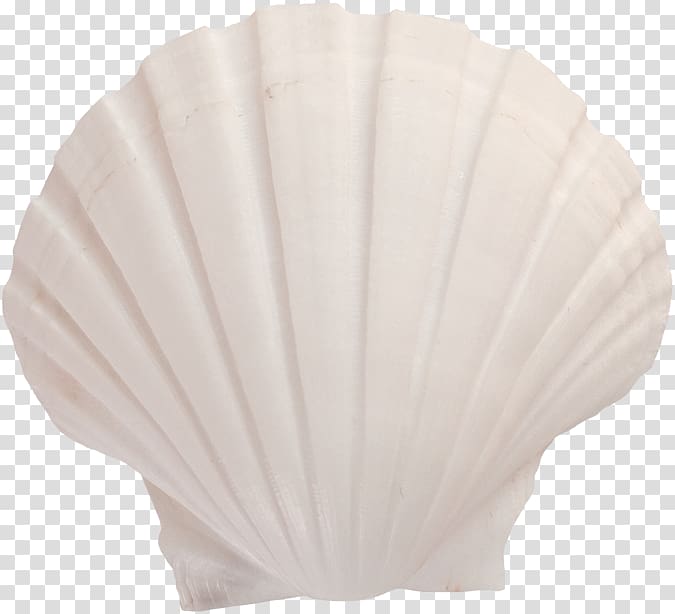The photograph showcases a large, clam-shaped, semi-circular white seashell prominently centered against a checkered light gray and white background. The checkers, small and squared, resemble the transparency grid used in Adobe Photoshop, suggesting a digital cutout presentation. The seashell features numerous deep grooves and ridges that extend from its squared bottom to its rounded top, giving it a textured appearance. These ridges are more pronounced towards the top where they fan out, while the bottom edge has jagged lines with two triangular flaps on each side. A slightly lighter line runs horizontally across the ridges on the rounded part of the shell, adding subtle detail to its otherwise plain design. The overall image combines the detailed natural form of the seashell with the modern, minimalistic background, highlighting its intricate structure.